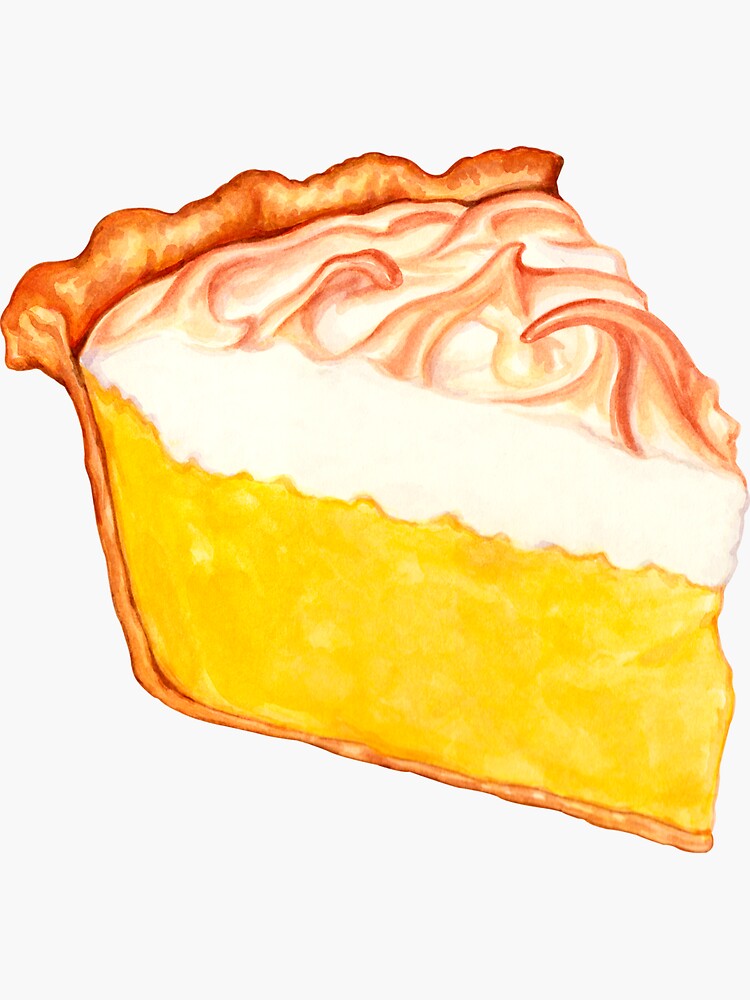In this image, there is a watercolor drawing of a vibrant, bright yellow pie slice. The pie features a thin, golden brown crust that extends towards a larger, thicker edge at the back. The creamy topping is white with brownish-toasted swirls, giving it a lightly caramelized appearance. The pie slice is angled, with the point facing the bottom right corner of the image. The background of the painting is a very light gray, enhancing the contrast and vibrancy of the yellow filling and the golden crust. The overall appearance of the pie slice is delicately detailed with a wavy texture on the cream, making it look incredibly appetizing.